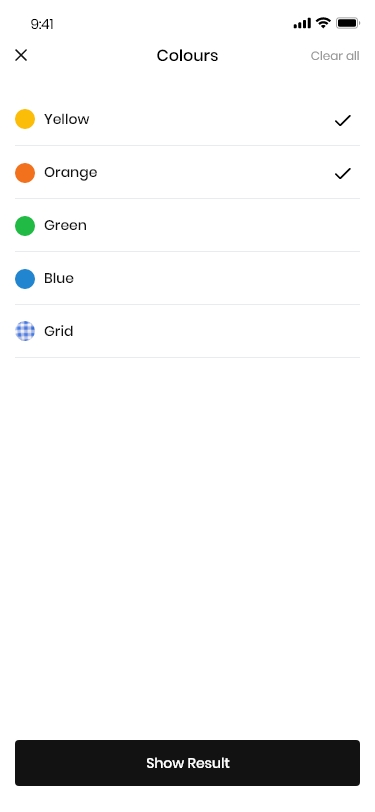The image appears to depict a mobile phone screen exhibiting a settings page specifically for color selection. At the top of the screen, the status indicators show a nearly full battery, active Wi-Fi, full signal bars, and the current time of 9:41 AM. The header of the settings page prominently reads "Colors." Below this header, a list of color options includes yellow, orange, green, blue, and a "Grid" option. Each color is represented by a dot in the corresponding color to the left of its name, with yellow and orange being currently selected. These color options are each displayed on individual lines. 

To the right of the "Colors" header, there's a "Clear All" button, and to the left, an "X" icon allows the user to close the menu. Beneath the "Grid" option, there is a large blank white space, which likely serves as a preview or additional setting area. At the very bottom of the screen exists a prominent black button labeled "Show Result," suggesting a functionality to apply or preview the selected color settings on the cell phone.